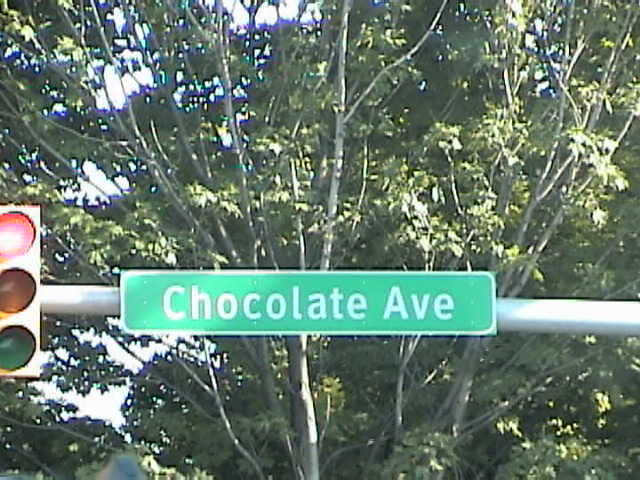The image depicts a green rectangular sign with a white border and white text that reads "Chocolate Avenue," mounted on a silver pole. The sign is quite narrow and features an uppercase 'C' for Chocolate and an uppercase 'A' for Avenue. To the left of the pole is a traffic light with three bulbs: red, amber, and green, with the red light currently illuminated. Dominating the background is a large tree with sprawling branches covered in green leaves, occupying most of the image. The photo is somewhat blurry, but the details of the sign and traffic light are discernible, making the primary elements of the scene clear despite the overall lack of sharpness.